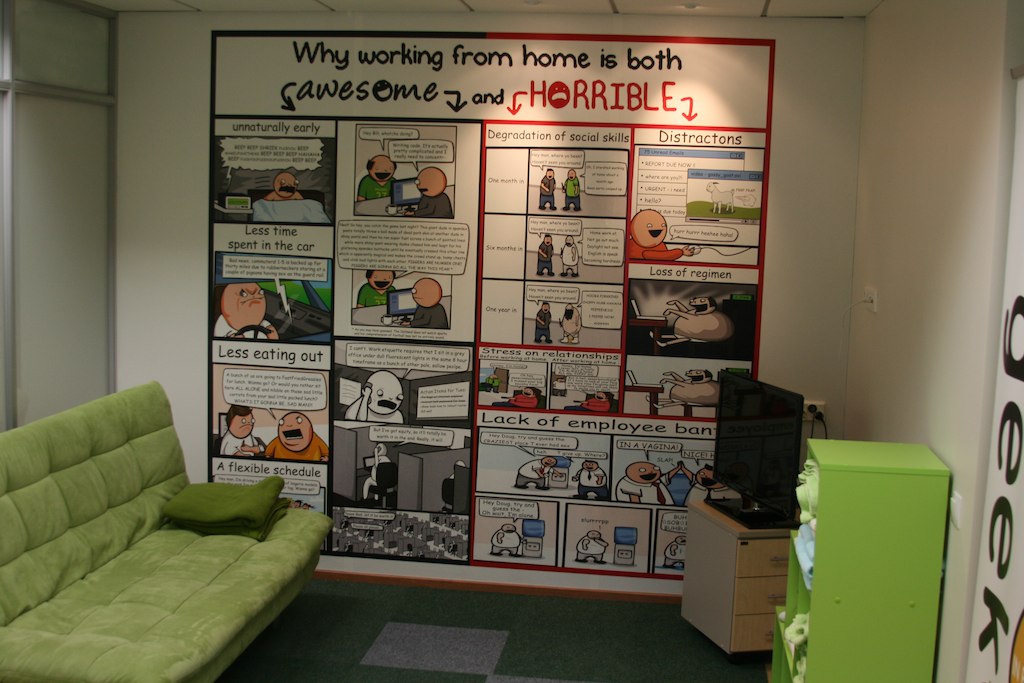This image captures a small, cozy room featuring a vibrant comic strip prominently displayed on the white wall. The comic strip, titled "Why Working from Home is Both Awesome and Horrible," features various cartoon characters with round heads and pink faces, depicting scenes that highlight the pros and cons of remote work. Some readable captions include "Unnaturally Early," "Less Time Spent in the Car," "Less Eating Out," "A Flexible Schedule" on the positive side, and "Distractions," "Loss of Regimen," "Deregulation of Social Life," "Stress on Relationships," and "Lack of Employee Banter" on the negative side.

In the bottom left corner of the room, there is a green couch draped with a darker green blanket. To the right, a small wooden shelf holds a black TV, and next to it is a green container filled with towels. The room features green carpet flooring with a light gray square in the center, tying together the room's peaceful yet eclectic ambiance. The room could be interpreted as a bedroom, living room, or a cozy home office, but the central focus remains the colorful and detailed wall comic that humorously critiques the experience of working from home.